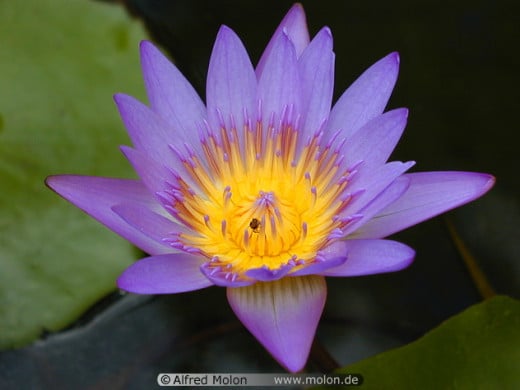This image showcases a vibrant purple flower with a radiant yellow center, predominantly resembling a daisy or water lily. The petals exhibit a gradient, transitioning from a light purple to darker shades at the edges, while the bright yellow center captures immediate attention. The flower is prominently centered in the frame, set against a stark, dark background which makes its colors pop vividly. Surrounding the flower are a few green leaves, with a lighter leaf on the left and darker ones in the other corners. An insect can be seen nestled within the yellow center, adding a touch of realism to the otherwise seemingly staged photograph. At the bottom of the image, the photographer's name, Alfred Molon, is inscribed along with his website, www.molon.de, indicating the image's authenticity and professional composition.